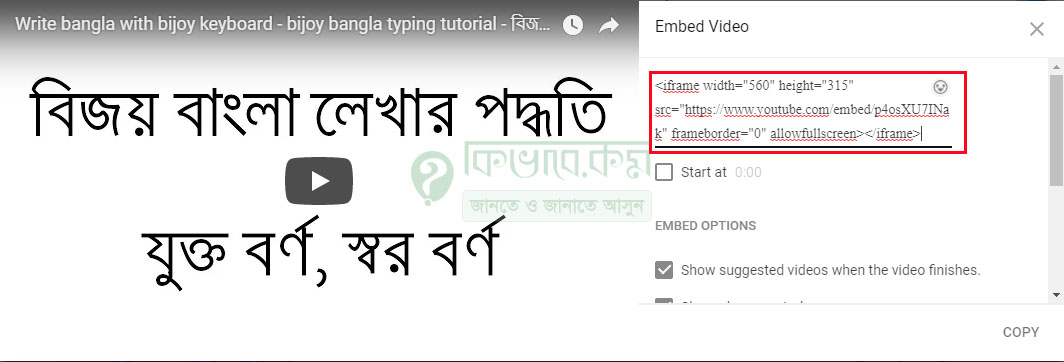The image is a detailed screenshot, likely from a YouTube video. The left side of the screen features a video with the title "Write Bangla with ByJoy Keyboard - ByJoy Bangla Typing Tutorial," displayed in white letters at the top. Below the title, there is text in another language. In the center of the video player is a gray play button with a white triangle indicating play. On the right side of the image is a section for embedding the video. This section fades from gray to white and includes options in black text. Specifically, it says "Embed Video" on the left side, with a white square nearby, and an 'X' positioned to the right side for closing the section. Below this, within a red-bordered box, there is HTML code, reading "iframeWidth=560, height=315," indicative of the video embed code. Further down, there is a checkbox labeled "start at 0.00," and beneath that, another section labeled "Embed Options" with two checkmarked options. The image is predominantly white, gray, black, and red, and appears to be a screenshot taken from a web browser displaying both the video and its HTML embed options.